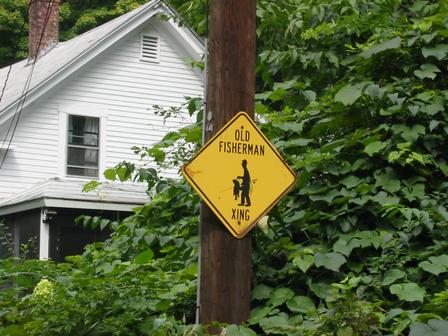The photograph captures a diamond-shaped yellow sign with a black border reading "Old Fisherman X-I-N-G." The centerpiece of the sign features a black silhouette of an older man walking with a fishing pole in one hand and a fish in the other. This sign is affixed to a brown utility pole. The background is lush with greenery, including ivy and large green leaves. On the left side of the image, there is a white, two-story farmhouse with a brick chimney on the top left, a covered porch, and a window with white curtains. Some foliage, including a light green flower, surrounds the porch and adds to the verdant setting.